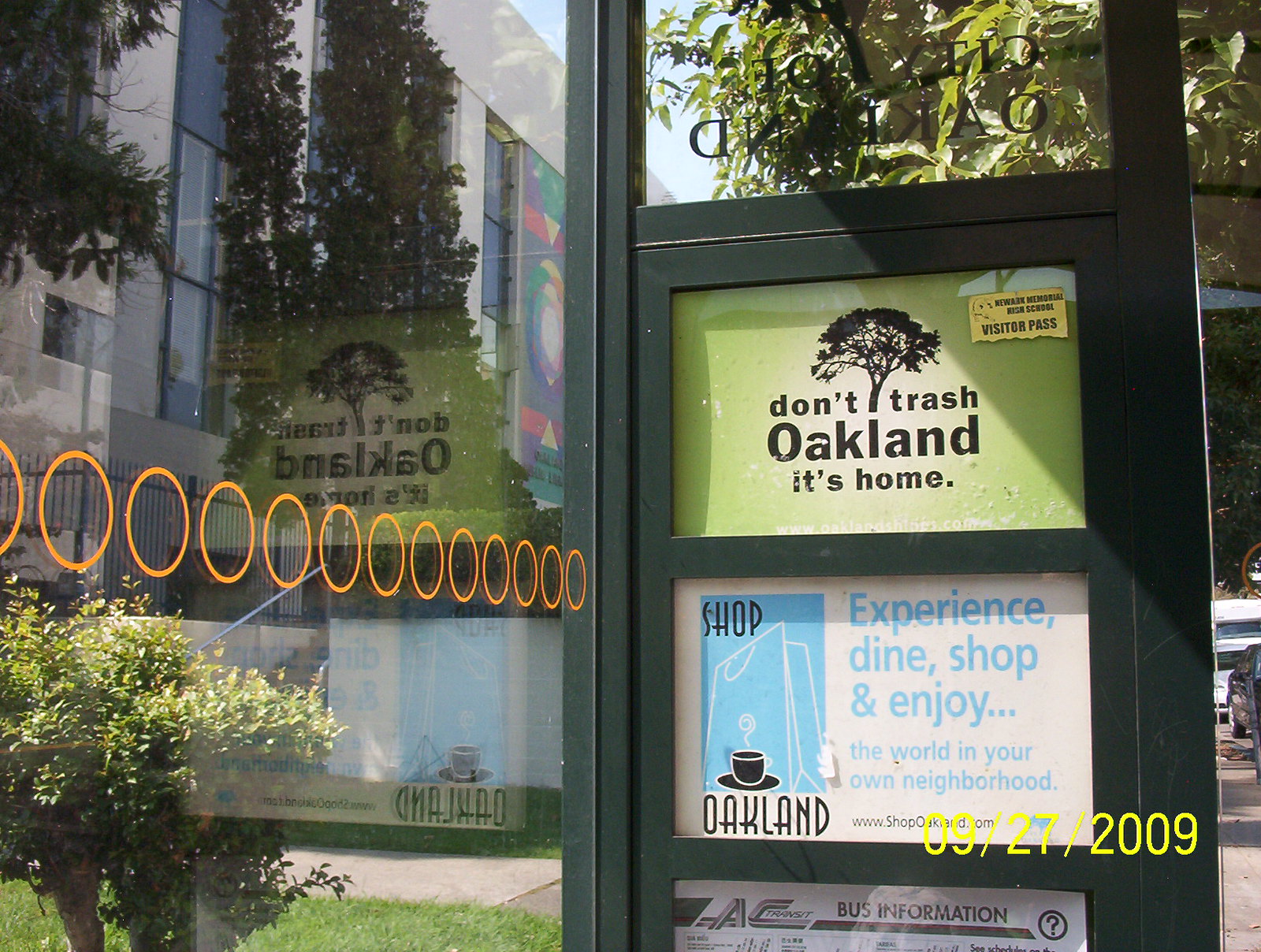This image, taken on September 27, 2009, features a glass or plastic side of a building in Oakland, California. Running vertically along the center of this glass or plastic surface are numerous yellow circles. To the left, the reflection in the material captures tall buildings and a small shrub or tree along with patches of grass on the sidewalk. The right side of the image showcases a series of rectangular black boxes featuring advertisements. The top box displays a picture of a tree with the text, "Don't trash Oakland. It's home." Below that is a blue and white box promoting local engagement with the message, "Experience, Dine, Shop, and Enjoy the World in Your Own Neighborhood." The bottom box provides "AC Transit, Bus Information." There is also a hint at "Shop Oakland" alongside imagery of coffee, suggesting nearby dining or retail options.